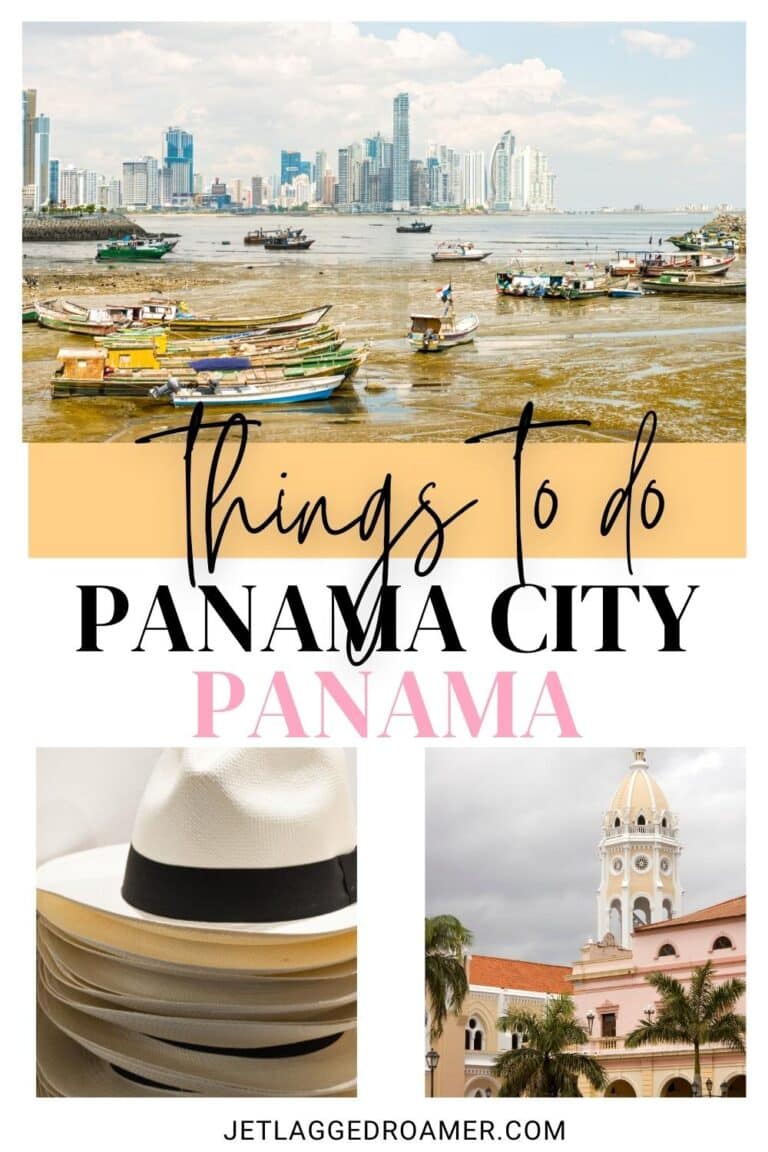**Caption:**
"Front page of a website showcasing 'Things to Do in Panama City, Panama.' The header image features a bustling waterway with a backdrop of the city's modern skyline beneath partly cloudy but blue skies. Numerous fishing boats, typical of local residents rather than wealthy yacht owners, occupy the waterway. Below this image, the central section highlights 'Things to Do in Panama City, Panama' in prominent text. To the left is a vibrant image of a stack of traditional Panama hats, while to the right, a majestic cathedral surrounded by palm trees stands tall under a clear yet slightly cloudy sky. At the bottom of the page, 'JETLAGAROMA.COM' is displayed in bold uppercase letters, marking the website's name. The overall theme presents a mix of urban sophistication and local lifestyle, inviting visitors to explore the unique experiences Panama City has to offer."